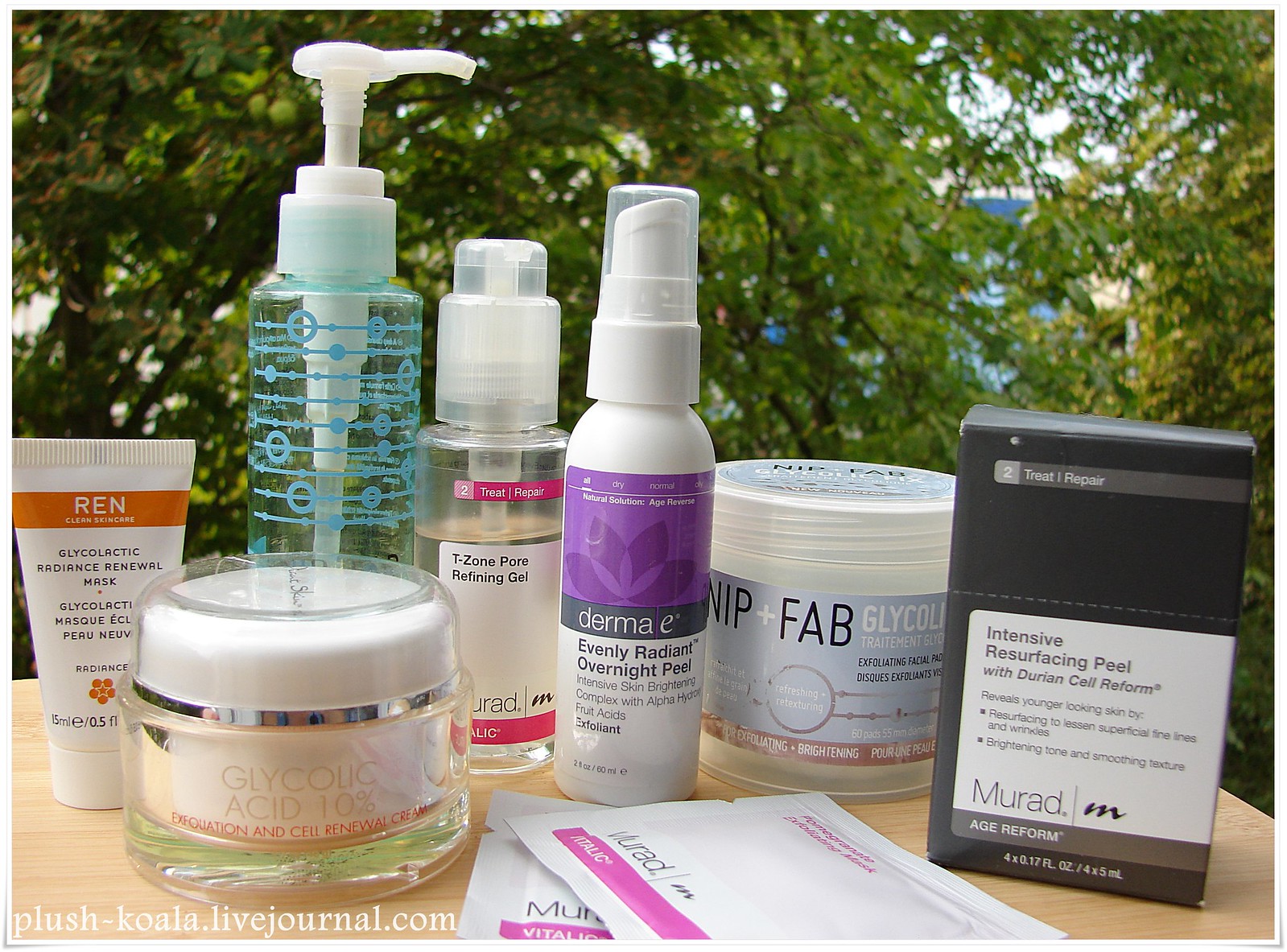In this image, a serene outdoor setting is depicted with an array of trees showcasing lush green leaves under a partly cloudy, blue sky. Through the foliage, the beige side wall of a nearby building is visible, accented with touches of blue. In the foreground, a light pinkish-brown table serves as the display surface for several beauty products. At the bottom of the image, the text "plushkoalalivejournal.com" is inscribed.

The beauty products include:
1. A black box labeled "Treat and Repair" featuring Murad's Intensive Resurfacing Peel.
2. A white jar with a light purple label from Nip + Fab, partially showing the name "Glyco..."
3. A white spray bottle with purple accents, identified as Derma E's Evenly Radiant Overnight Peel.
4. A product referred to as T-Zone Pore Retiring Gel.
5. A tall bottle adorned with blue circles.
6. A jar containing a pink substance with a white cap.
7. A small white tube.

Each item is meticulously arranged, creating a tranquil yet detailed composition that combines the natural environment with modern self-care elements.